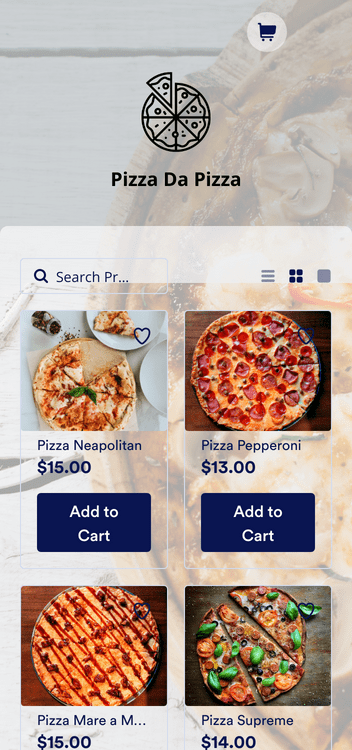### Detailed Caption:

This vertical image appears to be a screenshot or a screen grab from a website, possibly captured on a computer or a smart device. The background features a faded picture of a pizza, creating a subtle backdrop that does not overpower the foreground elements. 

In the upper-right corner, there is a white circle icon containing a gray shopping cart, which would typically display the number of items the user intends to purchase. 

At the center of the image, an icon of a pizza is depicted with one slice being partially removed. Directly below this icon, the text "Pizza Da Pizza" is prominently displayed in bold font.

A white horizontal separator divides the top section from the bottom. Beneath this separator, towards the lower left, a search bar featuring a magnifying glass icon allows users to search for items. To the right of the search bar, there are three icons arranged horizontally, though their specific functions are not detailed in the description.

The lower portion of the image lists various pizza options, each overlaid on the faded pizza background. These options include:

1. **Pizza Neapolitan** - Priced at $15, with an "Add to Cart" button.
2. **Pizza Pepperoni** - Priced at $13, with an "Add to Cart" button.
3. **Pizza Margherita** - Though partially obscured by "dot dot dot," it is priced at $15 and includes an "Add to Cart" button.
4. **Pizza Supreme** - Priced at $14, with an "Add to Cart" button.

This carefully designed layout emphasizes the menu and shopping cart functionalities while maintaining a consistent pizza-themed aesthetic.